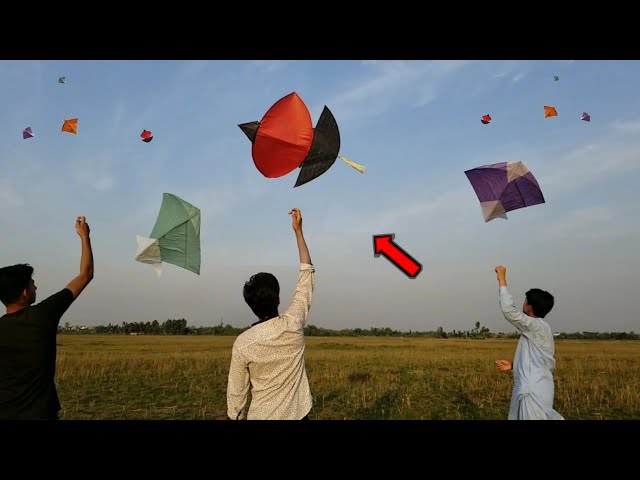This photograph captures an outdoor scene during a kite festival, bordered by a black header and footer that span the width of the image. The photograph itself, measuring approximately three inches in height and five inches in width, is divided into distinct sections. 

The top two-thirds of the image showcase a light blue sky with white cloud accents, possibly indicating afternoon transitioning into evening. Multiple colorful kites of various shapes and sizes are flown across this expansive sky, predominantly at the top left and right. Dominating the lower one-third of the image is a field of yellow grass, suggestive of dry conditions, bordered along the horizon by a row of dark green trees.

In the foreground, with their backs to the camera, stand three men with light brown skin, each raising an arm to fly their respective kites. On the left is a man with dark hair, wearing a black T-shirt, directing a mint green diamond-shaped kite with a smaller white diamond piece at the bottom. Centered in the image, another man with black hair is donned in a white button-down shirt with sleeves rolled up; his kite has a unique design consisting of a black triangular nose, a large red oval body, and a black semicircular tail with a yellow tassel. On the right, the third man, dressed in a light baby blue shirt, flies a predominantly purple diamond-shaped kite accented by smaller silver diamonds.

A prominent feature of the image is a red arrow with a black outline, placed between the center and the right men, pointing towards the distinctively designed black and red kite flown by the man in the middle. This detailed composition highlights the festive atmosphere and the engaging activity of kite flying under a serene sky.